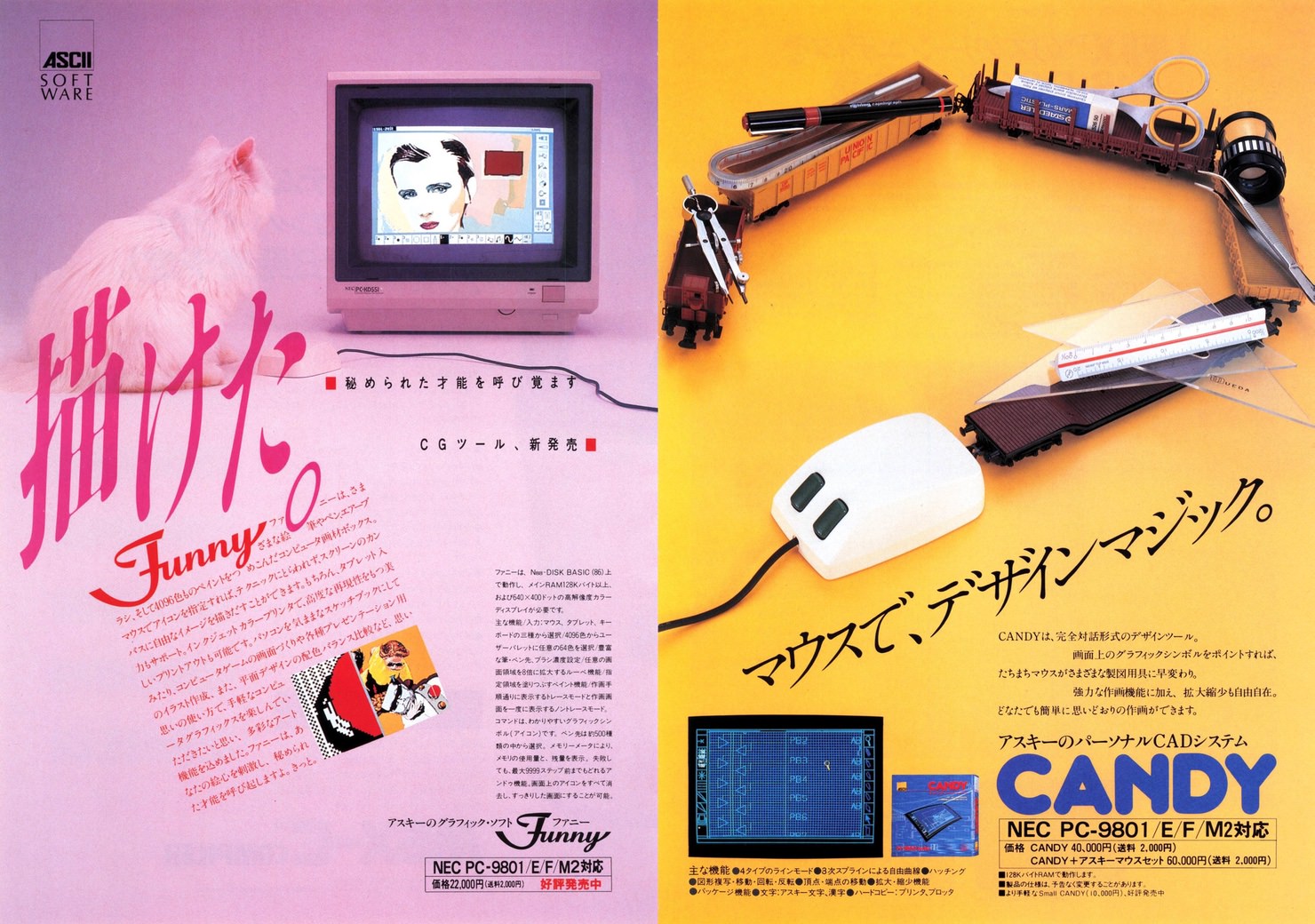This image, reminiscent of a 1980s magazine advertisement, is split into two distinct parts. On the left side, set against a pinkish-purplish backdrop, there is a retro-themed ad featuring a computer screen displaying a graphic image of a heavily made-up woman with an 80s new wave look. A white cat sits next to a mouse, intently watching the screen. The ad includes mostly Japanese text, though the word "funny" is prominently featured in red, and the brand "ASEH software" appears at the top left.

On the right side of the image, the background is a bright yellow, hosting an intricate arrangement of office supplies fashioned into a train. The makeshift train begins with an old-fashioned white computer mouse with a black cord, followed by various items like a ruler, tweezers, film, staples, scissors, a pen, and a compass. The train is arranged in a semi-circle and appears to be moving towards the bottom middle of the page. Below this whimsical construction, there's more Japanese text, accompanied by an English word, "candy," written in blue letters. A small rectangle featuring blue hues sits at the bottom left of this ad. Both sections of the image evoke a sense of nostalgia with their vivid colors and retro elements.